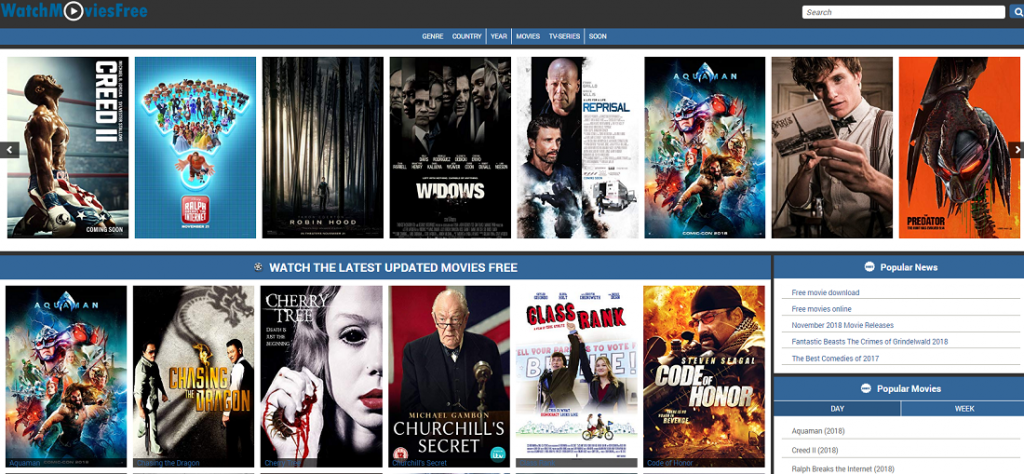The image appears to be a screenshot from a streaming platform, possibly Peacock, featuring a library of horror movies. The header says "Watch Movies Free" in blue and black bands, followed by the subtitle "Watch the Latest Updated Movies Free." The selection includes 14 different films, such as "Cherry Tart," "Creed 2," "Widows," "Glass Bank," "Church's Secret," "Code of Honor," and "Chasing the Dragon." The screenshot displays a visually striking array of colorful movie thumbnails, creating a vivid mosaic of horror genre options. The platform offers a plethora of recently updated films, beckoning viewers to explore its chilling collection.